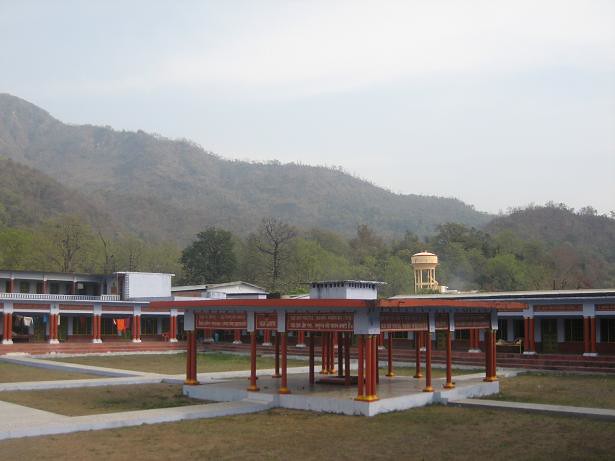The image showcases a serene outdoor scene, likely set in an Asian landscape, with a detailed view of a courtyard flanked by a mountain range in the distance. A prominent feature in the center is a gazebo comprised of red metal posts with gold bases, supporting a flat, possibly red, rooftop. The courtyard itself is interspersed with cement slabs and patches of grass. Surrounding the courtyard is a rectangular building with red pillars, possibly with a red and white facade, that reflects the gazebo's architectural style. Pathways connect the gazebo to various structures around it, creating a network of sidewalks leading in different directions. Further in the background, a light yellow water tower with a metallic or steel frame stands against a backdrop of densely forested mountains clad in brown and green foliage. The sky overhead is predominantly blue with scattered, mostly flat, white clouds. The overall scene, captured during the daytime, is infused with a tranquil ambiance typical of traditional Asian landscapes.